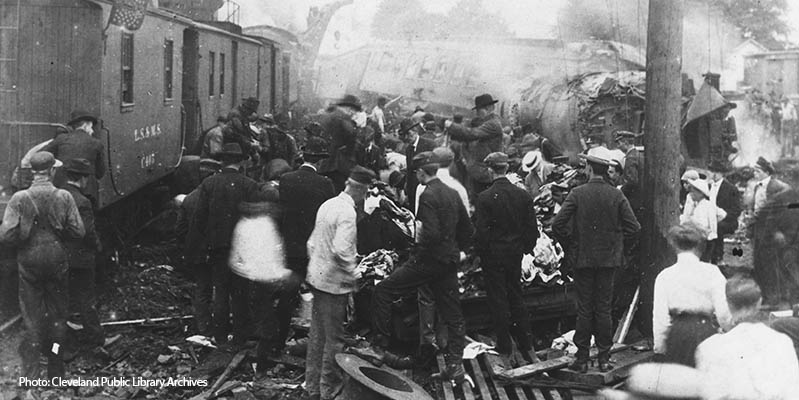The black and white photograph, captioned "Photo: Cleveland Public Library Archives" on the bottom right, depicts a chaotic and tragic scene from the aftermath of a train wreck. The accident appears to have taken place in Cleveland, possibly in the mid-1800s to early 1900s, as suggested by the period clothing of the men and women present. On the right side of the image, a severely damaged train is visible with its front completely smashed. In contrast, a train on the left appears to be relatively unscathed. A crowd of people, both men and women, can be seen frenetically moving about the scene, their attire characterized by hats and suits typical of the era. They seem to be engaged in rescue efforts, perhaps removing debris to help any survivors. The backdrop includes a smoky haze, enhancing the sense of urgency and tragedy. A pole stands to the right, behind which various metallic debris is scattered. The black and white tones of the photograph heighten the somber mood, emphasizing the shades of grays, whites, and blacks that capture the seriousness of the accident.